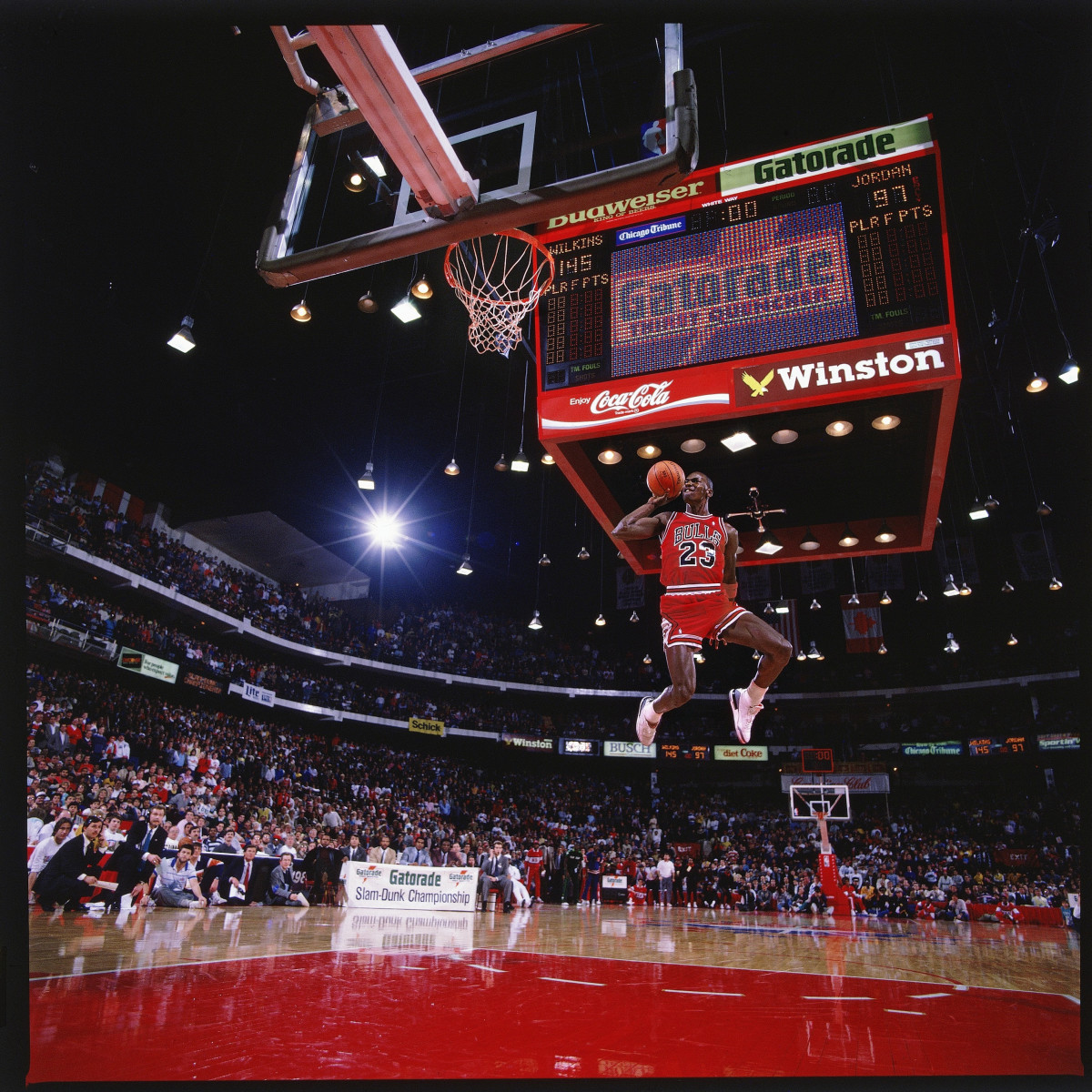This photo captures an iconic moment during a Chicago Bulls basketball game. The stadium is packed with spectators, fully engaged in the action unfolding before them. The central figure in the image is none other than Michael Jordan, in his prime, executing a breathtaking leap several feet off the ground. He's poised mid-air, wearing a red Chicago Bulls jersey emblazoned with the number '23' in bold black and white, and matching red shorts. The word "Bulls" stands out prominently on his jersey. In his right hand, he grips an orange basketball, on the verge of making a powerful dunk into the hoop positioned at the top of the frame. The tan court features a distinctive red square area, highlighting the iconic colors of the game. Above Jordan's head, a large jumbotron displays the logos of Coca-Cola, Winston, Budweiser, and Gatorade, further setting the scene in this electrifying moment in basketball history. No other players are visible on the court, emphasizing Jordan's standout performance as he soars through the air.